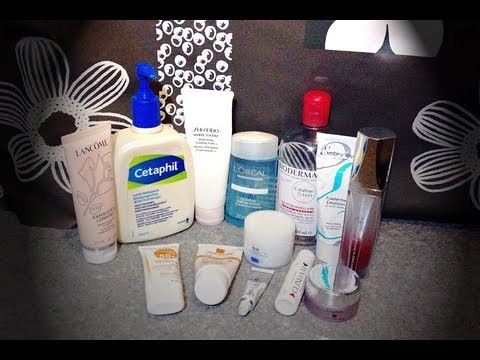In this image, a series of skincare products are carefully arranged on a gray countertop. The bottom section of the image features a black background transitioning into the flat gray countertop where the products are placed. In the foreground, two white bottles with orange labels lie on their sides. To the right of these bottles, there is a small tube followed by a cylindrical white tube. Further to the right is a wide jar with a purple base and a gray top. Above this jar, makeup items with a red and gray base and chrome caps are visible. Moving left, a white bottle with a mint green line can be seen, next to a larger white bottle with a red cap. Continuing left, there's a blue container with a white cap labeled "L'Oreal." A taller white bottle is positioned further left, adjacent to a container with a pump on top, labeled "Cetaphil," featuring a blue background with a white and green logo. To the extreme left is a light pink and white bottle. The backdrop of this arrangement is a dark brown wall adorned with two white floral designs, adding an elegant touch to the display.